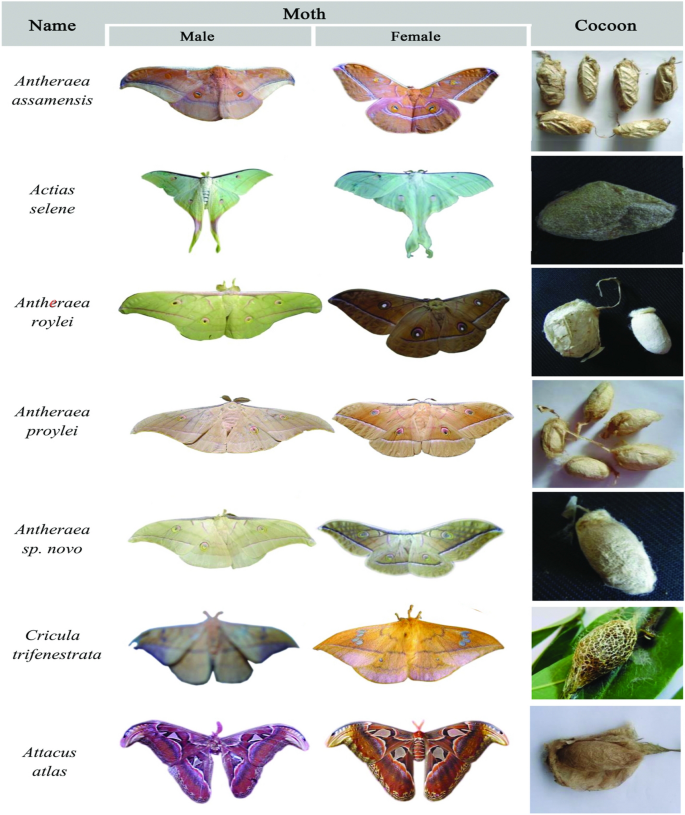The image depicts a detailed chart of seven different species of moths, showcasing vibrant and unexpected colors. Each species is represented by columns displaying the male, female, and cocoon stages. The layout includes a title in Times New Roman font, labeling sections such as "Name," "Moth," "Male," "Female," and "Cocoon." The moths exhibit a prominent array of colors including pink, teal, lime green, peach, maroon, and black. On the left, the scientific names of the moths, such as Atticus Atlas and Anthurius Novo, are provided, adding to the scholarly tone of the image. The visual splendor and diversity of the moth colors challenge the common perception that moths are merely white or drab in appearance.